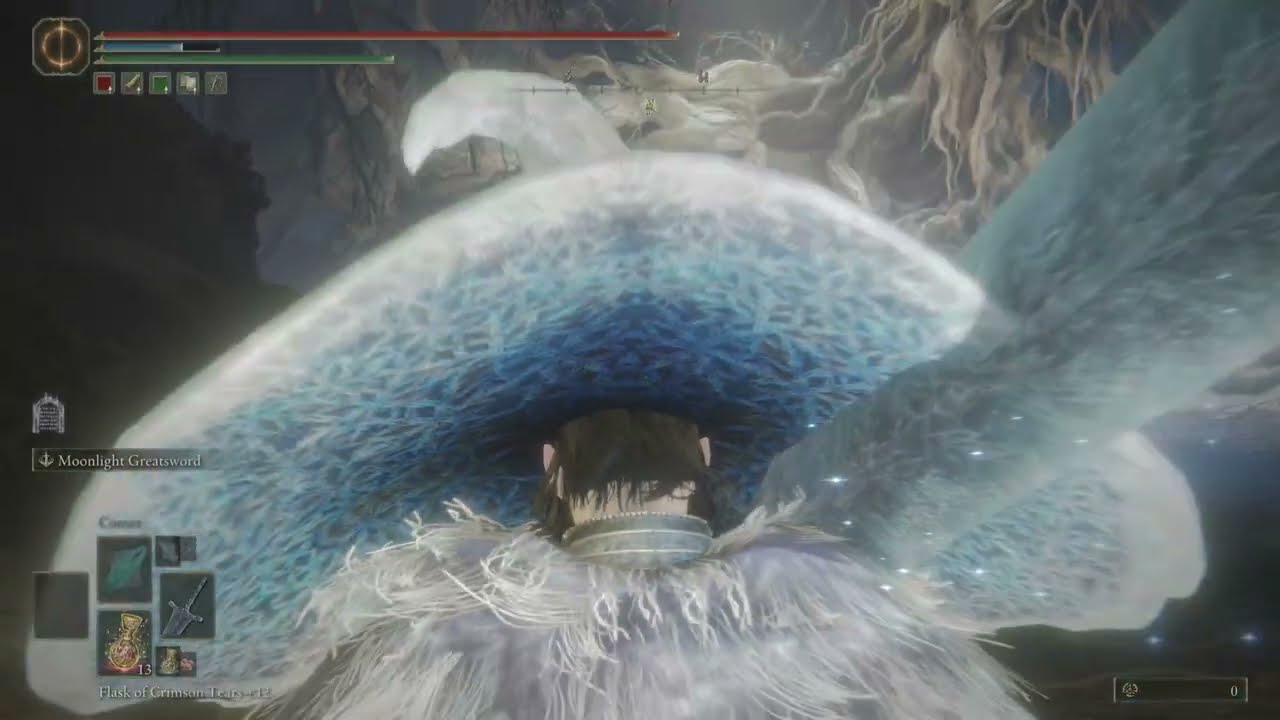The image is a detailed and ethereal screenshot from a video game. Dominating the foreground is a character whose back is turned towards the viewer. This character, most likely a man, has scraggly black hair and is adorned in an elaborate outfit with a gray, feathery high collar, and a dramatic, white, fur-lined cape. A large blue hat, resembling a mushroom with white edges and a gradient from light to dark blue, sits atop his head.

In the middle to top section of the image, there is an enormous, fantastically-colored mushroom cap that features many twisting, turquoise blue tree roots sprawling across its surface, creating a path-like design. The character appears to be standing or heading towards a cavernous or canyon-like environment with a mystical and dream-like ambiance, highlighting snake-like white clouds and a significant rock formation to the left of him.

The edges and corners of the image are filled with typical video game interface elements. The upper left corner displays red, green, and blue progress bars, a compass with a "W" for west or wind, and tiny symbolic blocks denoting possible actions or attributes. Controls for character manipulation, including a sword, appear in other corners, underscoring the gaming aspect. Text in the image is mostly unreadable but suggests the title might include "Moonlight." The scene has a whimsical and otherworldly quality, perhaps set in a fantastical frozen landscape.